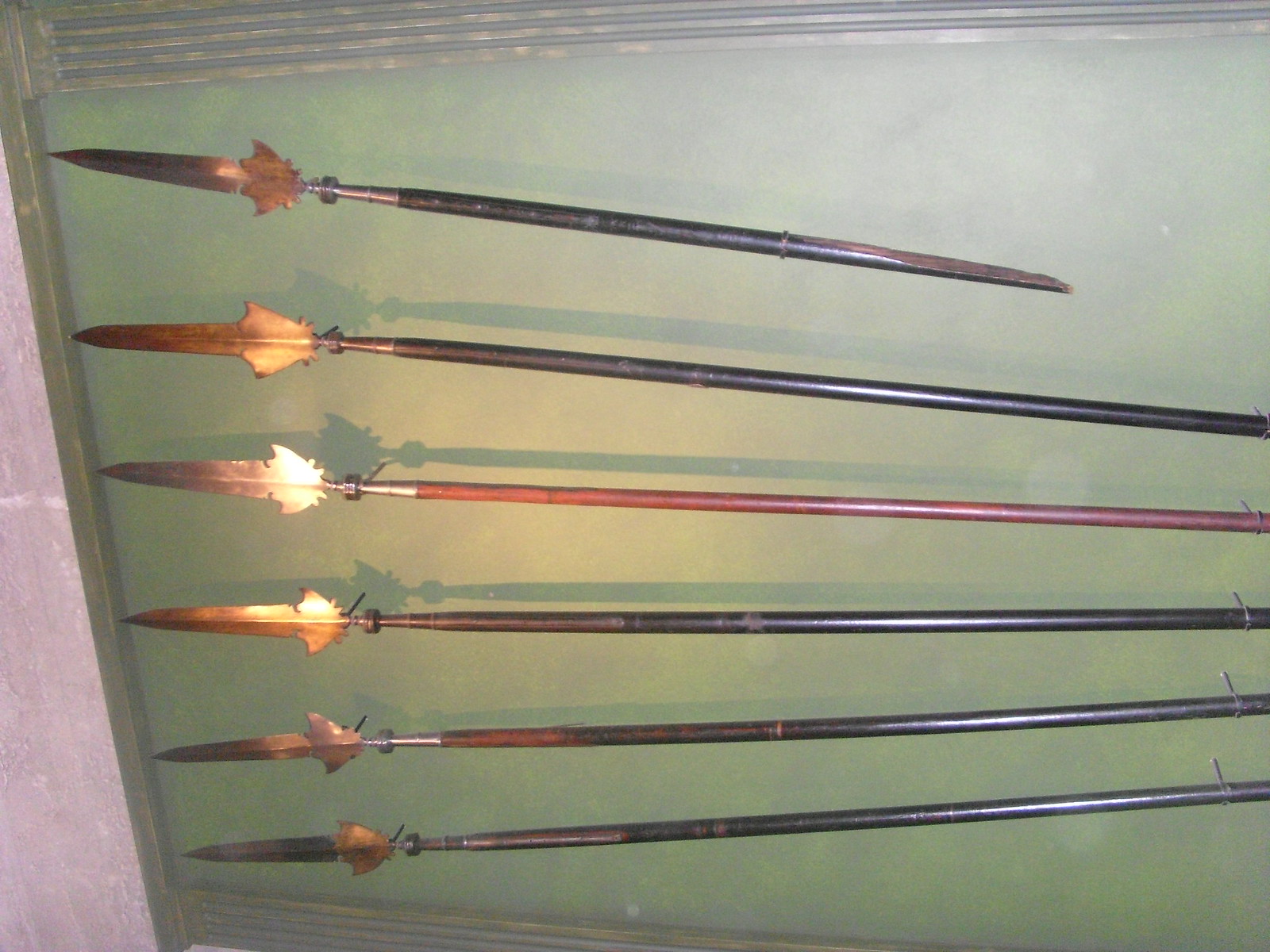This photograph features six spears meticulously displayed within a glass box. The spears are arranged horizontally, stacked in a vertical line with each spear aligned one above the other from top to bottom. The topmost spear features a black handle and is oriented with the handle pointing to the right and the metal tip to the left. This spear appears damaged, with its wooden shaft broken in half. The second spear has a longer black handle with a similar golden-colored metal tip. The third spear down shifts to a brown handle, maintaining the same golden tip as the previous ones. The bottom three spears share a black-brown handle and identical golden-colored tips. Each spear's tip resembles a knife with a leaf-like metal structure extending from the blade, forming a singular piece of steel. The metal tips are connected to slender wooden shafts, evoking a vintage appearance, possibly from the 1700s. The spears are displayed on a bluish-white backdrop, enclosed in a wooden frame with shadows cast behind them, adding depth to the presentation.